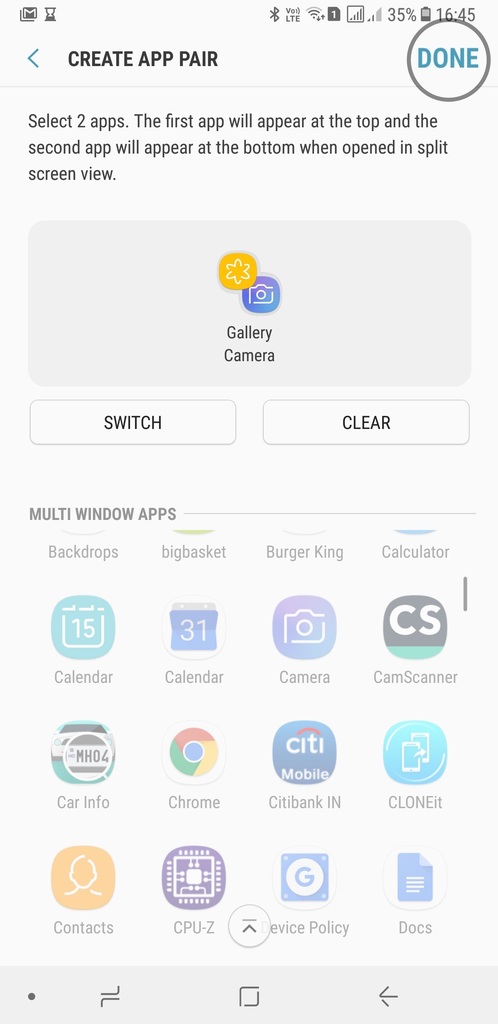Screenshot of a Smartphone Displaying Multi-Window App Management Screen

Top Left:
- Email icon.
- Sand timer icon, indicating time has elapsed (sand at the bottom).

Top Right:
- Array of status icons including Bluetooth, LTE, Wi-Fi, and others.
- Document icon with the number "1".
- Bar graph icon depicting signal strength (2 out of 3 bars).
- Battery icon indicating 35% charge.
- Time displayed as "16:45".

Central Area:
- Below the time display, a gray-outlined circle with blue "Done" text inside.
- Opposite, a blue left-pointing arrow with black "CREATE APP PAIR" text in capital letters.

Main Section:
- Gray horizontal separator.
- Two lines of descriptive black text.
- Below the text, a gray rounded-corner rectangle housing two icons:
  - Yellow icon with a white star.
  - Purple icon with a white camera outline.

Bottom Section:
- Two white buttons with gray outlines labeled "SWITCH" and "CLEAR" in capital letters.
- Gray horizontal line labeled "MULTI-WINDOW APPS" nearby.
- Array of application icons listed underneath.